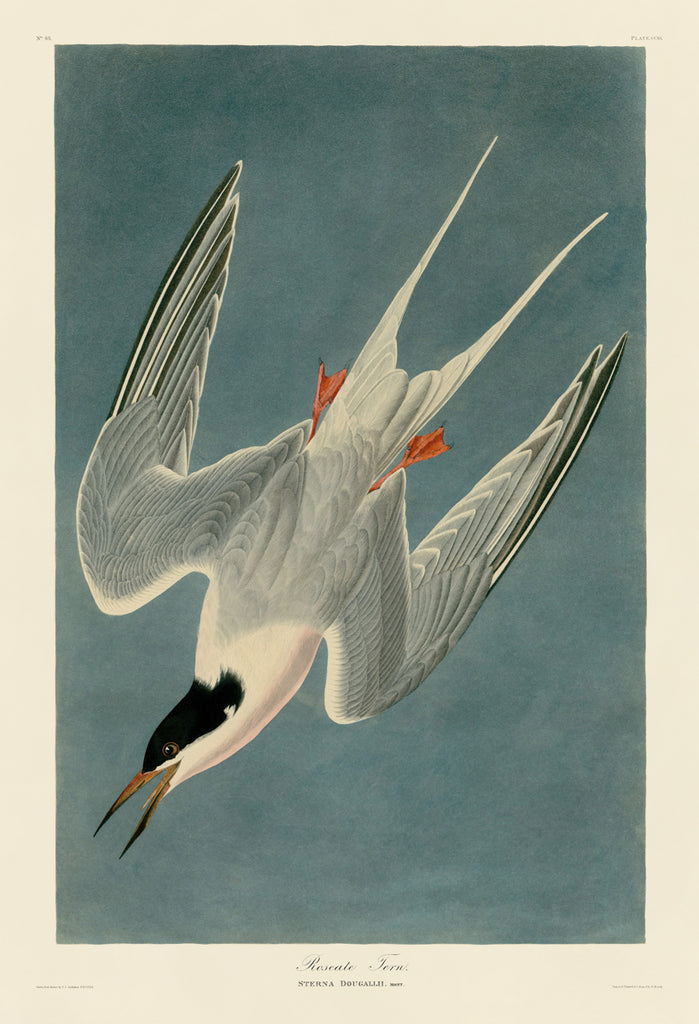The image depicts a beautifully detailed drawing of a bird diving from the sky, set against a gradient background that transitions from darker blue at the top to a lighter, creamy off-white around the edges. The bird, captured in mid-flight, is angled diagonally from the upper right to the lower left corner, displaying its striking features. Its long, pointed beak is orange with a black tip, partially open, and black feathers frame its eyes and head. The bird's white feathers, interspersed with black and light bluish-gray accents, extend outwards, showcasing a dynamic pose. The webbed feet are a vibrant orangey-yellow, tucked back as the bird dives. The poster-like image includes text at the bottom; in cursive, "Anturna Dugali" is prominently featured, with additional smaller black text on the lower portions that are hard to decipher. The meticulous details and careful coloration make this artwork a captivating illustration of avian beauty.